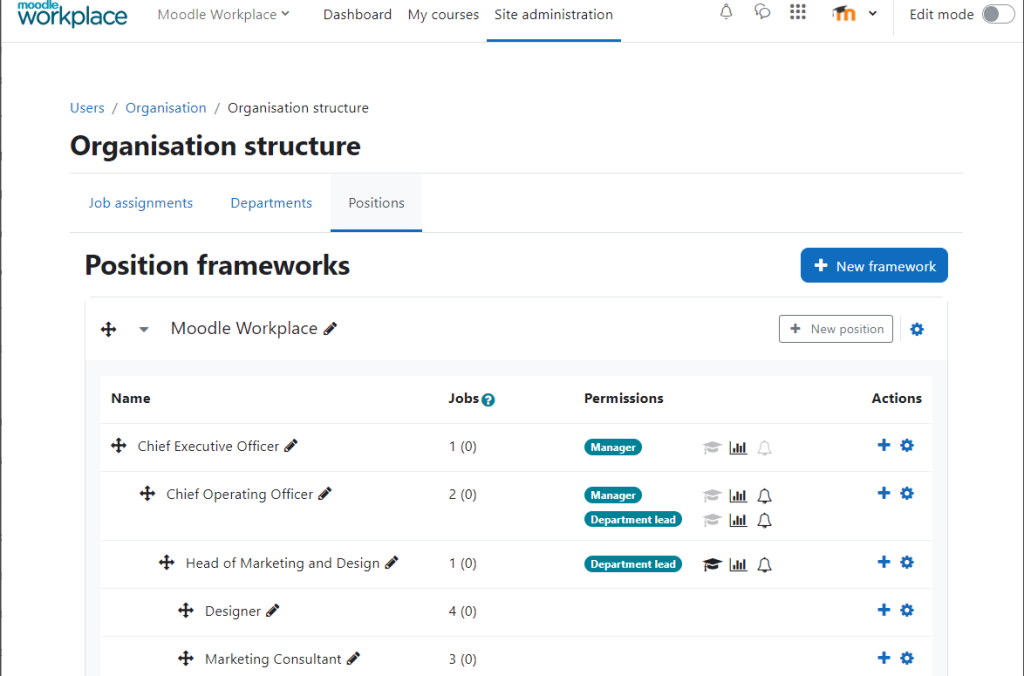The image captures a detailed screenshot of a Moodle Workplace web page interface. In the upper left-hand corner, the company name "Moodle Workplace" is prominently displayed. Adjacent to this is a drop-down menu featuring four main sections: Moodle Workplace, Dashboard, My Courses, and Site Administration, with the latter highlighted by an underlined blue line.

Beneath these primary headings, additional sections titled "Organization Structure" and "Position Frameworks" are shown, accompanied by a blue "New Framework" button. This suggests options for creating new organizational frameworks.

The interface is organized into multi-column tables with headings labeled Name, Jobs, Permissions, and Actions. Listed positions include Chief Executive Officer, Chief Operating Officer, Head of Marketing and Design, Designer, and Marketing Consultant. Next to these positions are small aqua oval buttons labeled "Manager" and "Department Lead."

Within the Actions column, each row features a blue plus sign and a blue settings button, indicating additional configurable options for each role. The main page is structured around headings for Job Assignments, Departments, and Positions, highlighting open positions within the Moodle Workplace organization.

The screenshot overall provides a comprehensive overview of the administrative interface for managing organizational roles and frameworks within Moodle Workplace.